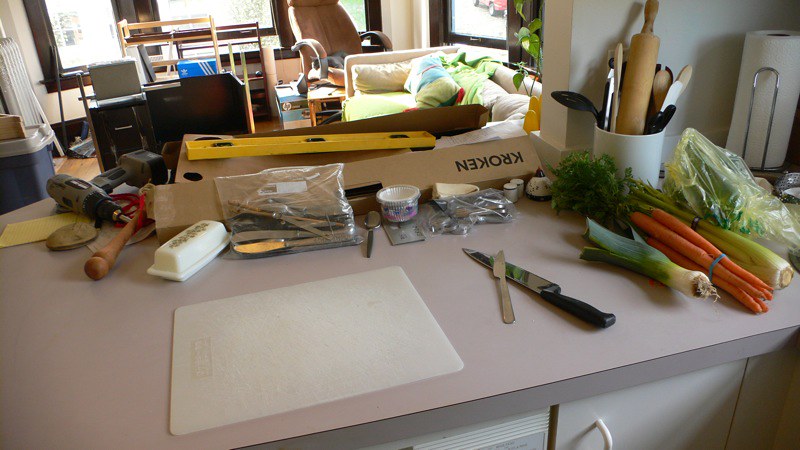The photograph showcases a slightly diagonal view of a kitchen countertop with a pinkish hue. Underneath, only a small portion of white cabinets is visible in the lower right-hand corner. Prominently placed on the counter is a well-used white cutting board, beside which lie a cutting knife and a kitchen knife. Further to the right are fresh vegetables: a bunch of carrots, celery, a leek, and some greens in a plastic produce bag from the grocery store. 

In the upper right-hand corner of the image stands a paper towel holder with white paper towels. To its left, a white holder contains an assortment of utensils including a rolling pin, wooden spoons, and plastic spoons. Moving further left, a drill is situated next to a long IKEA box labeled "KROKEN," likely containing a shelf. Atop this box rests a yellow level. In front of the box, a Ziploc bag holds several butter knives, and nearby, a butter dish and a cupcake holder container are visible.

The background reveals a glimpse into a living room complete with a couch, a chair, and windows that let in natural light, indicating a well-lit and homey environment beyond the kitchen.